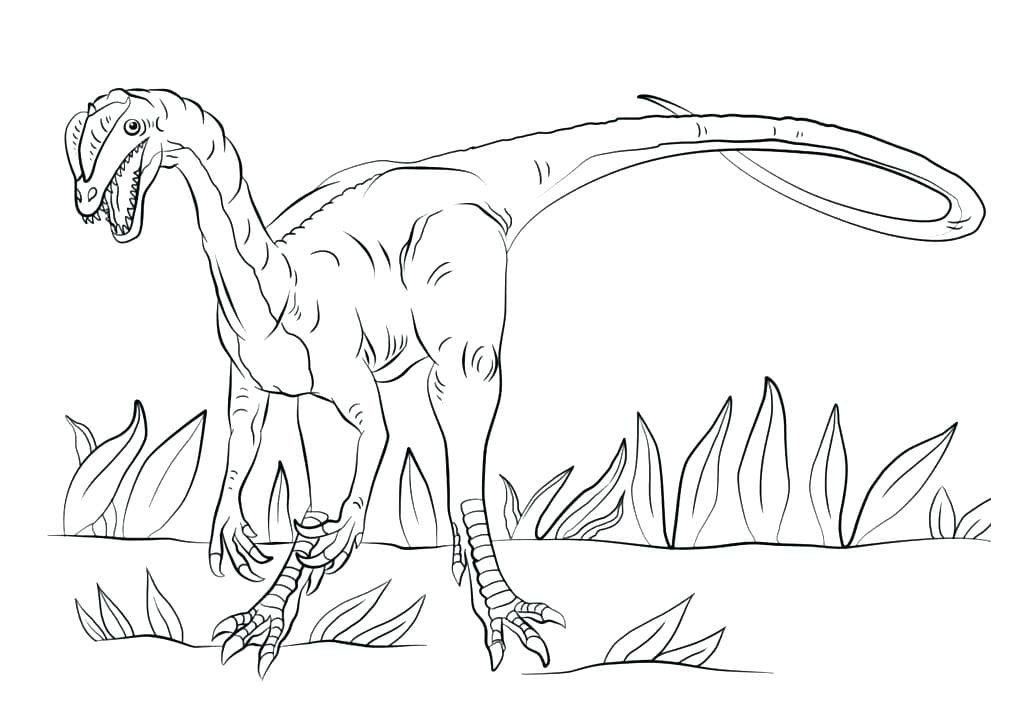This is a detailed pencil drawing of a dinosaur standing on two legs against a white background. The dinosaur, illustrated in black lines, exhibits a detailed array of features. Its powerful legs are muscular at the top and adorned with scales as you move down. Each foot ends with three sharp claws, poised menacingly above a flat surface scattered with leaves and plants. The arms, shorter and hanging down in front, possess four fingers each, all tipped with fierce claws. The creature's body tilts slightly to the left, and its long, sinuous neck curves gracefully upward before angling down into a wide-open mouth bristling with sharp teeth. Two simple dots represent its nose, and a black spot marks its eye, giving it a focused, predatory gaze. A lengthy tail extends to the right, initially winding downward before curling back up and then looping to the left. The ground below, subtly detailed with undulations, raises slightly in the background, adding depth to this prehistoric scene.